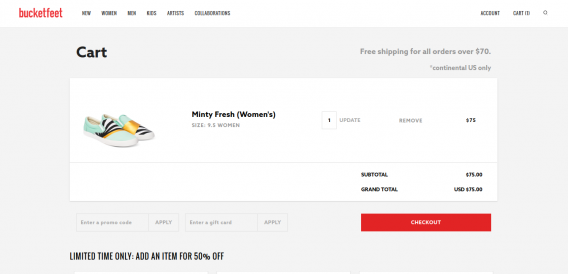This horizontally oriented screenshot captures the final page of a shopping cart where a customer is ready to complete their purchase. At the top left corner, the text "Bucketfeet" is prominently displayed in red, with navigation subcategories—New, Women, Men, Kids, Artists, and Collaborators—listed next to it. The top right corner features icons for Account, Cart ID, and a Search function.

The main portion of the screen consists of a white horizontal box over a light gray background, labeled 'Cart.' A key promotional message states, "Free shipping for all orders over $70 in the continental U.S. only." Within the cart, there is a photograph on the left showing a pair of stylish slip-on shoes with black and white stripes, accented by gold and light green. The shoes have a white plastic sole and are identified as "Minty Fresh Women's, size 9.5." Only one pair of shoes is selected, with each pair costing $75.

Further details include the subtotal and grand total of the purchase near the bottom. Two interactive fields are available for customers looking to redeem promotions or gift cards with "Apply" buttons next to each. To the lower left, a time-sensitive offer states, "Limited time only. Add an item for 50% off." Positioned at the bottom right corner beneath the grand total is a conspicuous red "Checkout" button inviting the user to finalize their purchase.